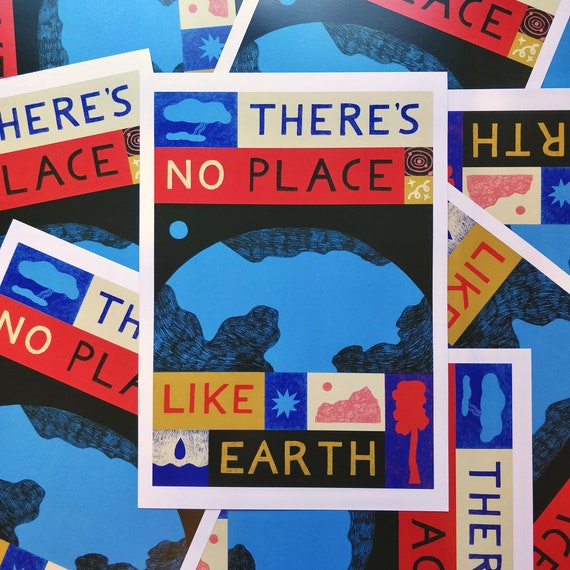The image is a digitally created collage resembling a flyer, repeated multiple times and scattered like a pile of overlapping posters. At the top center of the primary, perfectly upright flyer, large blue letters spell out "THERE'S NO PLACE," and at the bottom, red letters state "LIKE EARTH." The central drawing on the flyer shows the upper half of planet Earth, sketched in black pencil with blue oceans, resembling a child's drawing. Surrounding the Earth are several smaller boxes: one at the top left features blue clouds, another on the right displays a small red tree, a blue star, and a water droplet, all arranged on a dull-colored background. Some flyers are upside down or tilted in various directions, adding to the cluttered appearance. The entire collage is bordered in white, giving it a framed look.